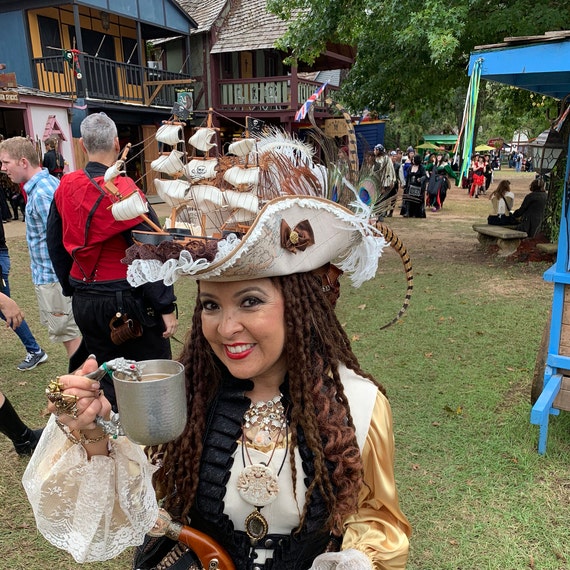The photo captures a lively scene at a semi-outdoor festival, likely a Renaissance Fair with a pirate theme. The central focus is a mixed-race woman with fair skin and long, dark brown braids, dressed in a cartoonish yet detailed pirate costume. She smiles broadly, showing her teeth, and salutes the camera with her right hand while holding an aluminum cup adorned with a skeleton hand in her left. Her elaborate hat, whimsically topped with a miniature pirate ship, adds a playful touch to her attire. She accentuates her look with jewelry, including rings and necklaces, and has a fake pistol tucked into her belt. The background reveals a bustling crowd, some in modern attire and others in period clothes, against a backdrop of blue and gray-green buildings, suggesting an event where attendees dress in themed costumes. The late afternoon sun casts a warm glow over the scene.